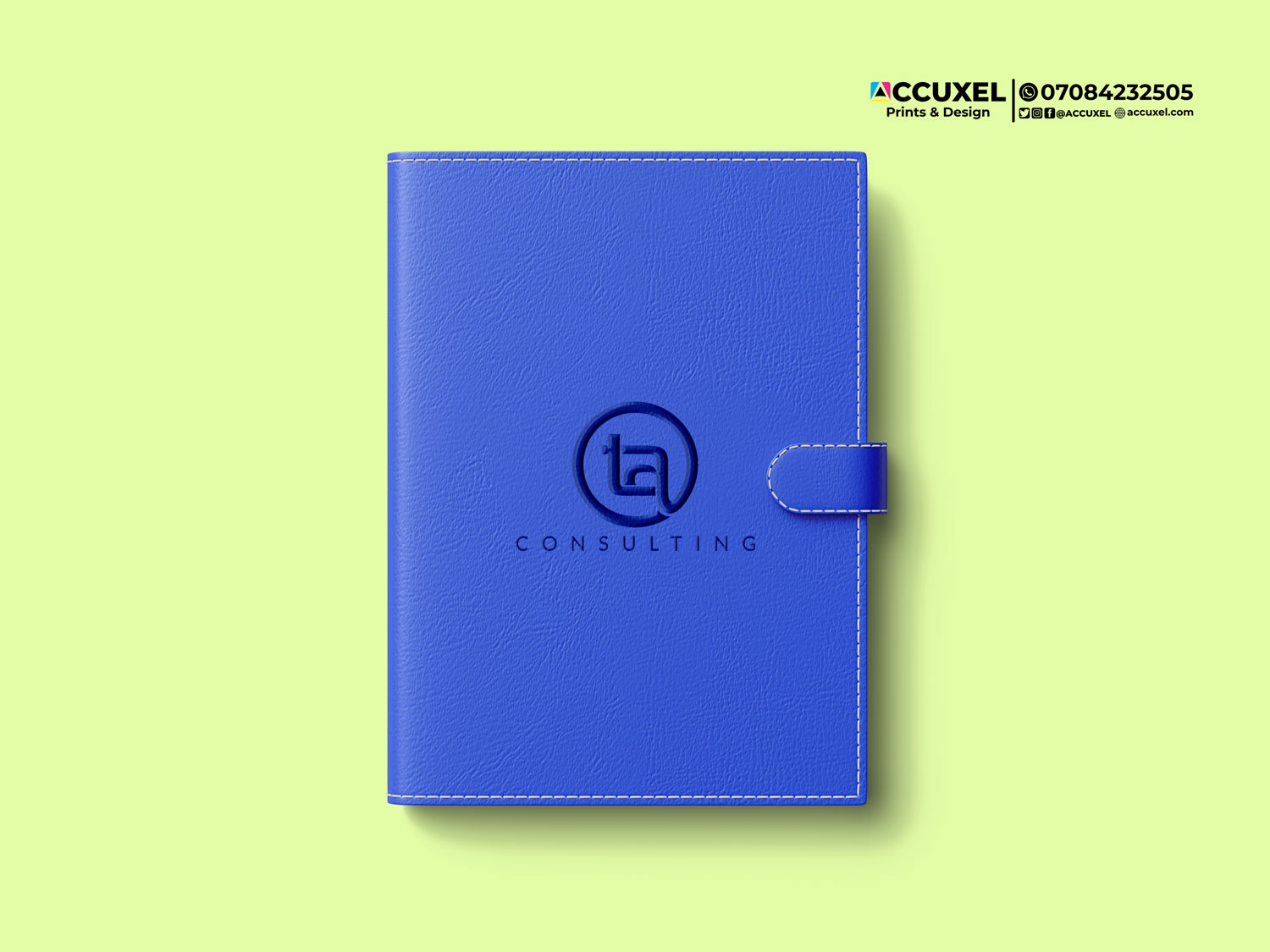The rectangular advertisement (wider than it is tall) has a pale neon yellowish background. At the top, it prominently features the company name "CCUXEL Princeton Design," followed by a phone symbol and the phone number "0708-423-2505," all aligned seamlessly. Adjacent to this, it mentions "accuxel.com." The upper section also includes small icons for Instagram, Twitter, and Facebook. Below this text, centrally positioned, is a blue leather journal with a magnetic flap on the right side for closure. The front of the journal is stamped with the word "Consulting" beneath a logo composed of a circle containing a square and additional lines, possibly forming the letters "T" and "A." The background color highlights the product, showcasing an example of the print and design services offered by AccuXel, particularly for office and business products.